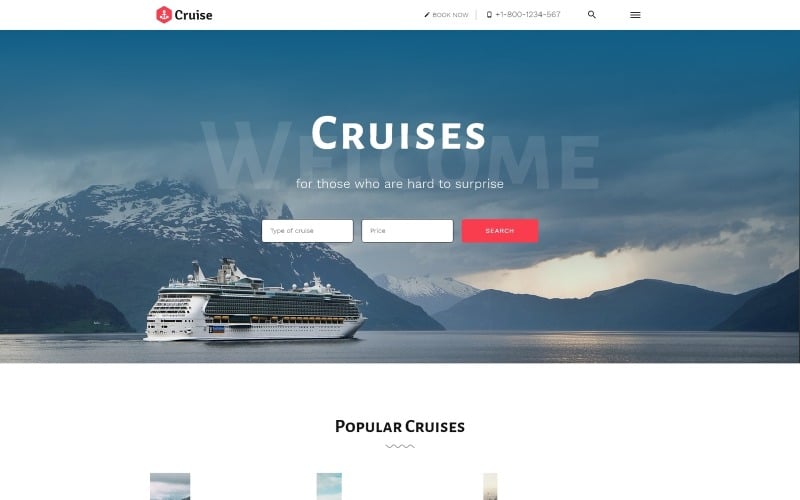This image, sourced from the website Cruz, displays a well-composed scene of both branding and natural beauty. On the top left corner, the brand "Cruz" is prominently featured in black print, with the 'C' capitalized and the remaining letters in lowercase. Adjacent to the brand name is a striking red hexagon emblem, which encloses a white anchor symbol, reinforcing the nautical theme.

The scene extends downward to reveal a magnificent cruise ship navigating a vast, tranquil body of water, resembling a serene lake or a broad waterway. In the background, rolling mountains add a majestic touch to the landscape. The sky overhead is adorned with an array of stunning, large gray clouds, interspersed with beams of sunlight piercing through, creating a dramatic interplay of light and shadow.

The cruise ship itself is grand and predominantly white. The deck is bustling with tall structures, indicative of various amenities and recreational facilities available to passengers. The ship’s bow prominently displays the word "Cruises," while a welcoming message, stating "Welcome" and "for those who are hard to surprise," can be seen faintly in the backdrop, suggesting an exclusive and extraordinary experience aboard this vessel.